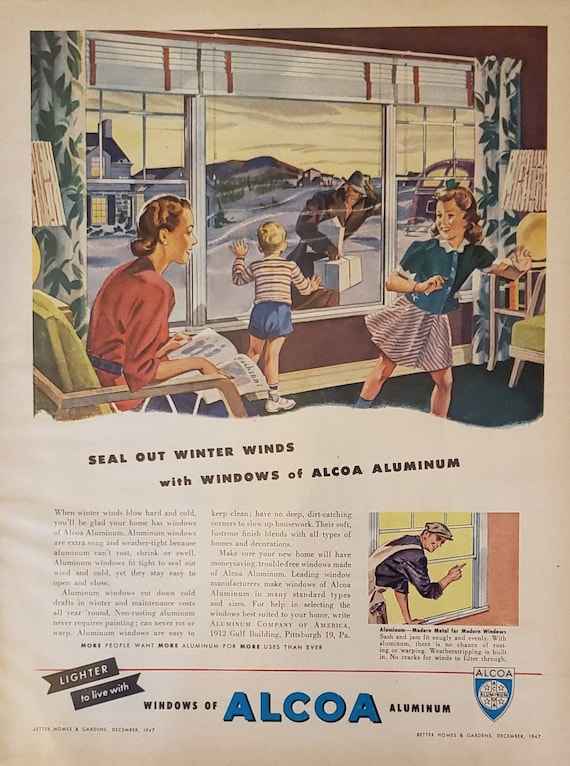This image, evocative of a mid-20th century magazine ad, features a nostalgic, weathered design that transitions from a brownish hue at the top to a light pinkish color, suggesting aged paper. Dominating the upper section is a charming illustration reminiscent of the 1950s, portraying a cozy family scene. A mother, seated comfortably in a chair, is engrossed in reading a magazine or book. Her two children are animated around her; the daughter seems to be looking at her mother while the son, dressed in shorts and a shirt, peers out of a large window. Outside, amidst a backdrop of snow and icy winds, a man—presumably the father—is depicted holding his hat, bracing against the gusts, and clutching a package. Wind streaks artistically emphasize the harsh winter weather.

Prominently displayed beneath the main illustration is the caption, "Seal out winter winds with windows of Alcoa aluminum," underscoring the advertisement's focus. Additionally, there's an extensive block of small text elaborating on the benefits of Alcoa aluminum windows. Adjacent to this text, a small inset image depicts a workman amidst the installation process of the windows. Near the bottom of the ad, a red line and a flag motif draw attention to the slogan, "Lighter to live with windows of Alcoa aluminum." The brand name "Alcoa" is presented in blue, accompanied by the company's logo, further reinforcing the product's identity and trustworthiness.